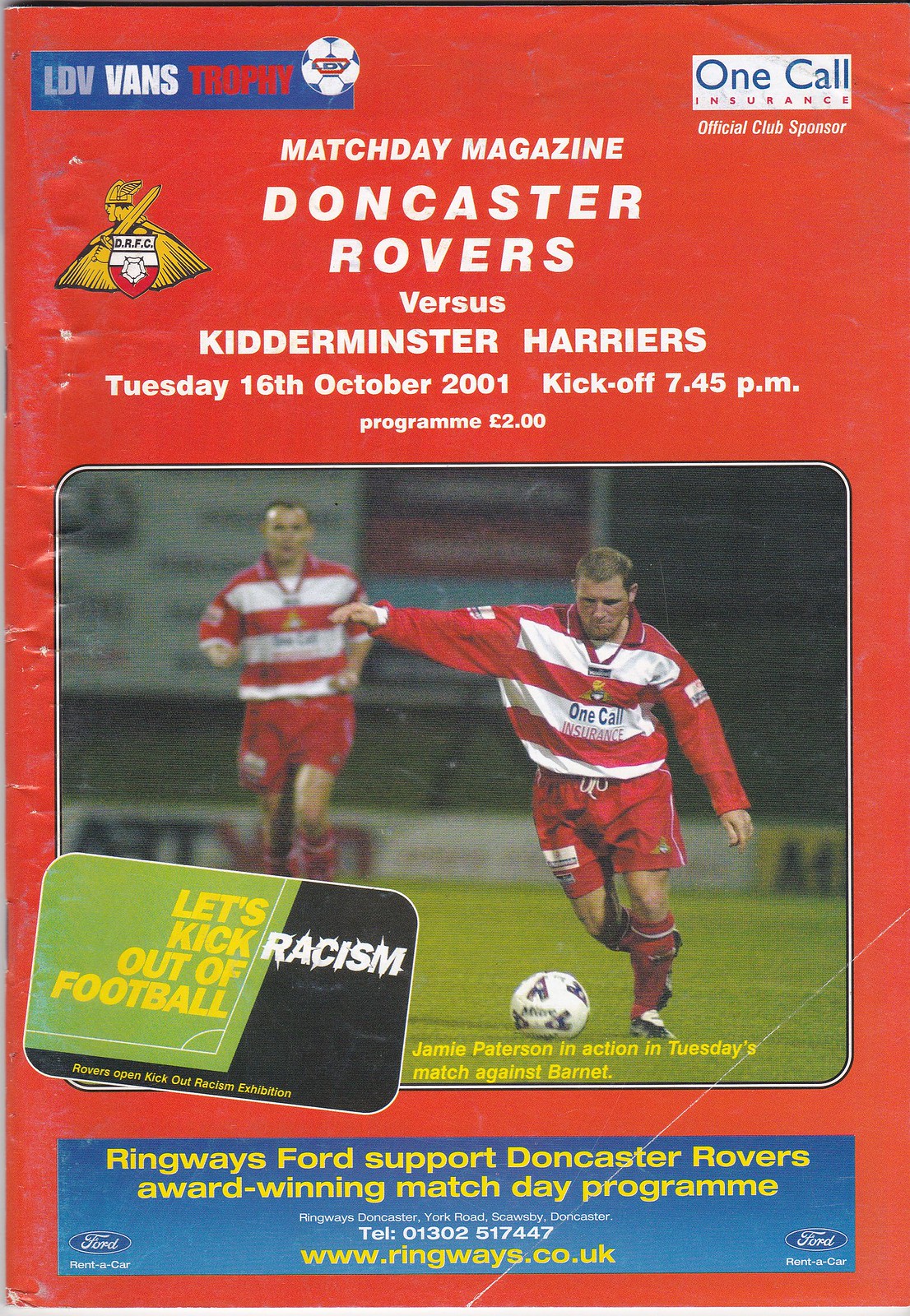The image is the front cover of a rectangular, portrait-shaped match day magazine for a soccer game. The background is predominantly red, with various text and logos. The centerpiece is a colored photograph of two soccer players on green grass, both in mid-action. One player, prominently in focus, is wearing a long sleeve red soccer jersey with a folded down collar and white stripes on the front, red shorts with a white stripe on the side, red soccer pads on their shins, and black and white soccer cleats. The other player is similarly attired in red and white. Below the photograph, in yellow font, it reads "Jamie Patterson in action on Tuesday's match against Barnett."

At the very top, in white font, it states "Match Day Magazine, Doncaster Rovers versus Kidderminster Harriers," alongside the date "Tuesday, 16th October, 2001" and the kickoff time "7.45 p.m." It mentions the price, "program two pounds." The upper left-hand corner features a blue rectangle with an LDV Vans Trophy logo along with a soccer ball. The upper right corner contains the text "One Call Insurance" in blue, acknowledging the official club sponsor. Adjacent to the top-center text is a gold emblem of a person with a hat and wings, accompanied by "DRFC" in white with red below it. An overlay on the photograph bears the slogan "Let's kick racism out of football." 

At the bottom of the cover is a blue bar with the Ford logo, promoting "Ringaways Ford support Doncaster Rovers, award-winning match day program,” followed by a phone number and website.